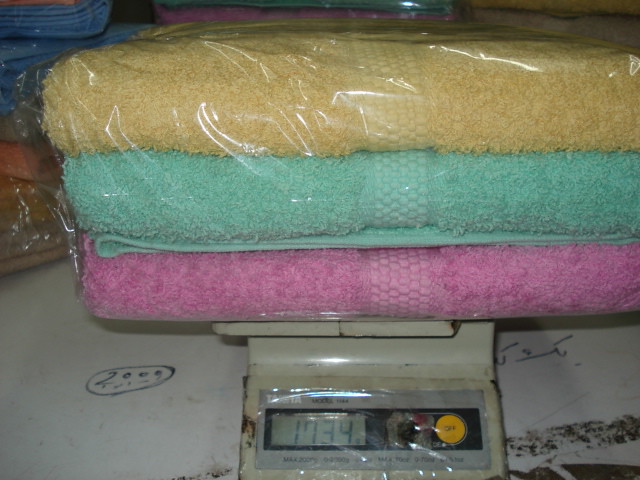This detailed image depicts a bundle of three neatly folded towels, each wrapped in plastic. The top towel is yellow, followed by a teal one, and the bottom towel is pink. All three are placed on an antiquated, off-white weighing scale, which displays a weight of 1,734 grams. The scale features a yellow 'off' button and shows signs of age, with a rusted surface and bubbled plastic over the display. This setup rests on an old, possibly basement countertop, which is marked by penned handwriting from 2009 on the left and various scribbles on the right. The countertop appears worn and dirty, suggesting a storage or moving environment. In the background, additional bundled sets of towels can be seen, emphasizing the aged and cluttered setting.